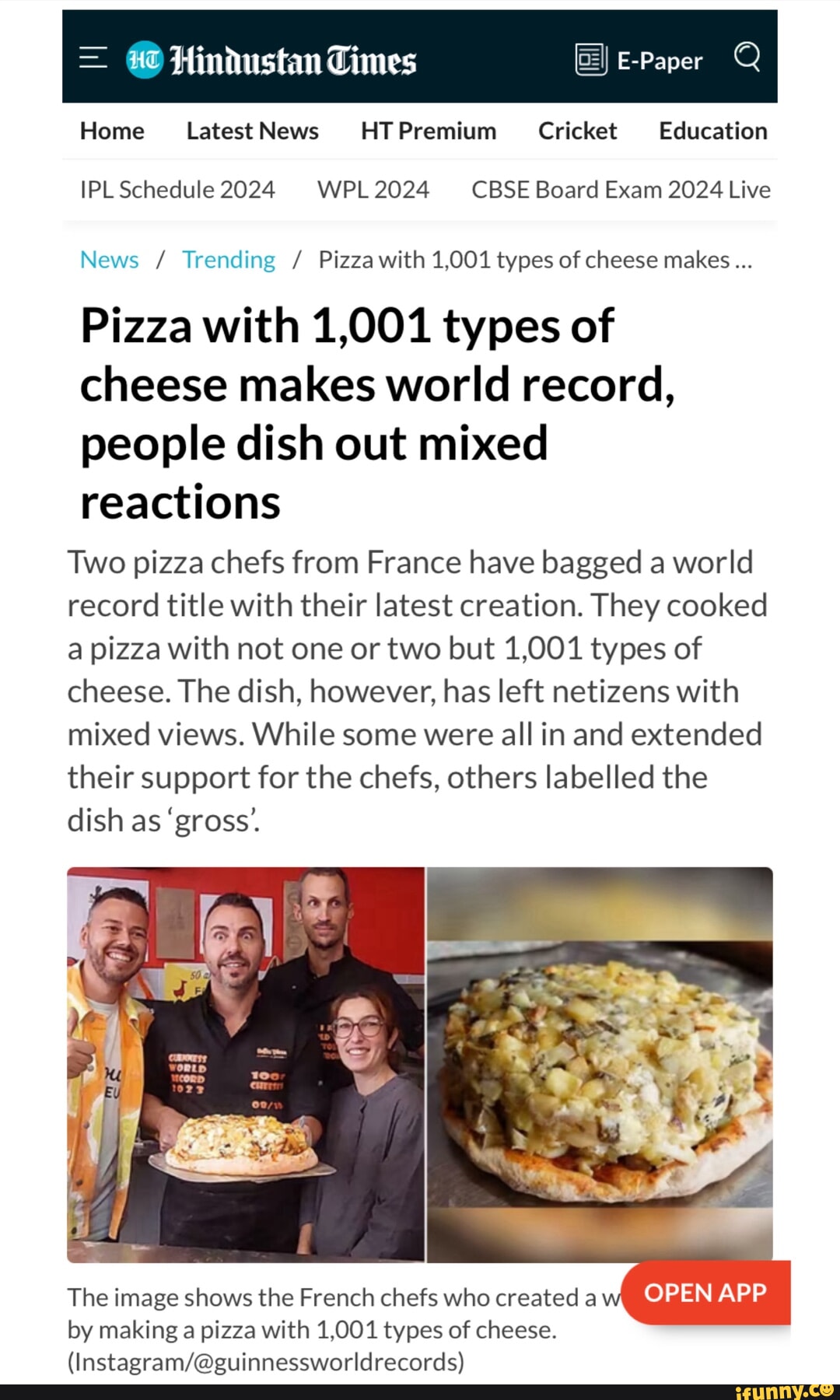This is a detailed caption:

The image is a screenshot of a portion of an article from the Hindustan Times, as posted on ifunny.com. The header of the webpage has a dark blue background. On the far left of the header, there is a white menu icon. Positioned to its right is the Hindustan Times logo, followed by an icon of a newspaper. Adjacent to this, "e-paper" is written in bold white letters. Further to the right, there is a magnifying glass icon.

Beneath the header, a horizontal menu features five categories: "Home," "Latest News," "HT Premium," "Cricket," and "Education." Below this menu, three specific links are highlighted: "IPL Schedule 2024," "WPL 2024," and "CBSE Board Exam 2024 Live." 

Continuing down the page, a navigational path reads "News / Trending / Pizza with 1001 types of cheese makes...", indicating the article's location within the website. The headline of the story is prominently displayed in large black letters, stating: "Pizza with 1001 types of cheese makes world record. People dish out mixed reactions."